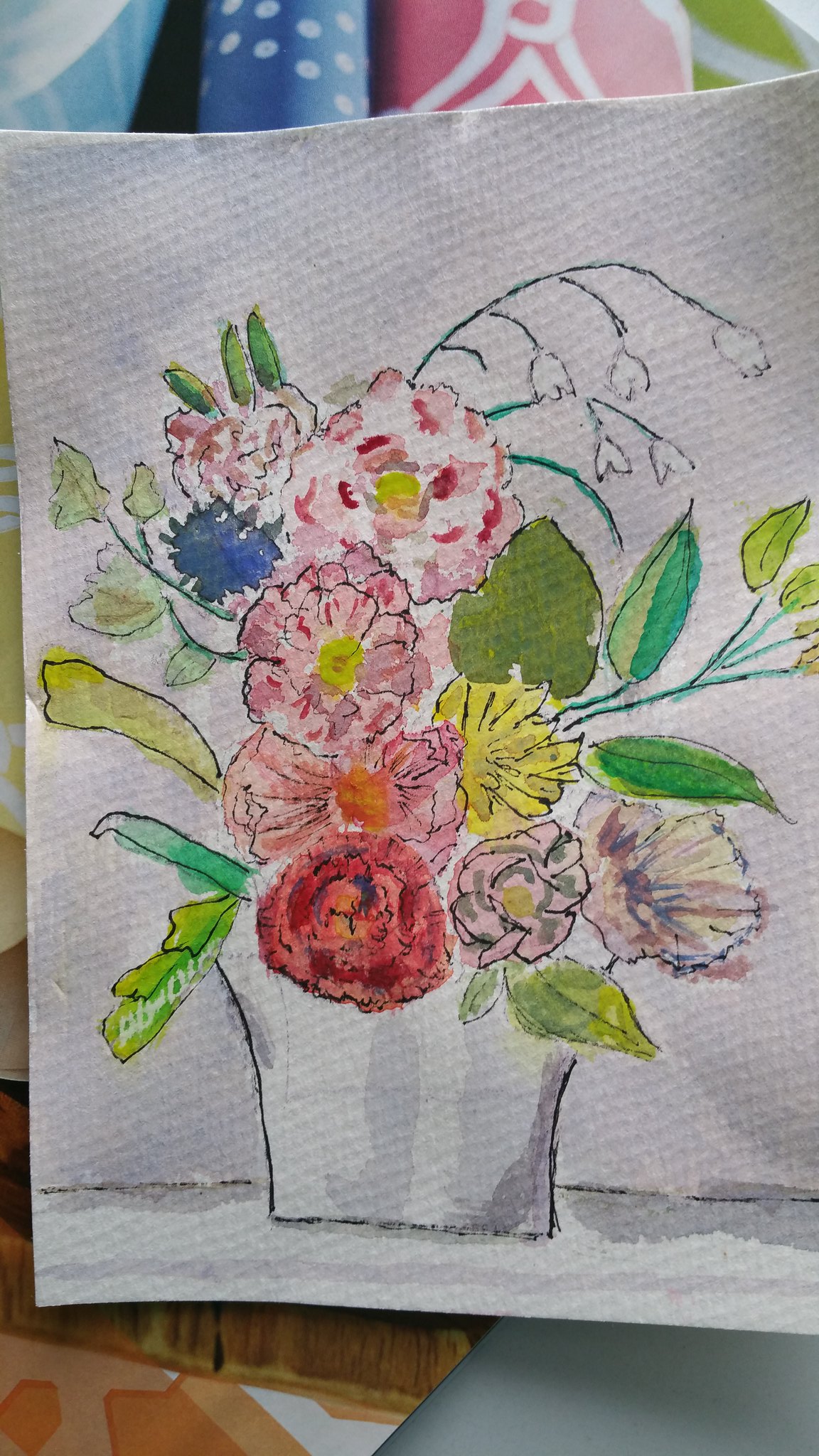In the background of the image, a vibrant array of patterns create a rich tapestry. On the left side, a section showcases blue fabric adorned with white dots transitioning into white lines set against a lighter blue background. Moving towards the right, there is a piece of cloth with red and white patterns, followed by an adjacent section of green and white designs. 

In the foreground, the focus of the image is a hand-drawn depiction of a pot brimming with flowers, set against a clean, white backdrop. The pot itself is white, providing a neutral base for the explosion of color above it. At the center bottom of the arrangement is a striking red flower, flanked by two pink flowers situated slightly higher. To the right of the red bloom, clusters of white flowers are interspersed with tiny yellow spots, adding a touch of warmth and variety.

Green leaves extend from the flower pot, framing the blossoms. Among these, there is a delicate, thin-stemmed flower that stands out for its slender structure. The assortment also includes flowers with wider petals that blend shades of white and pink. Overlooking the vibrant ensemble is a solitary purple flower, adding a final note of contrast to the colorful display.